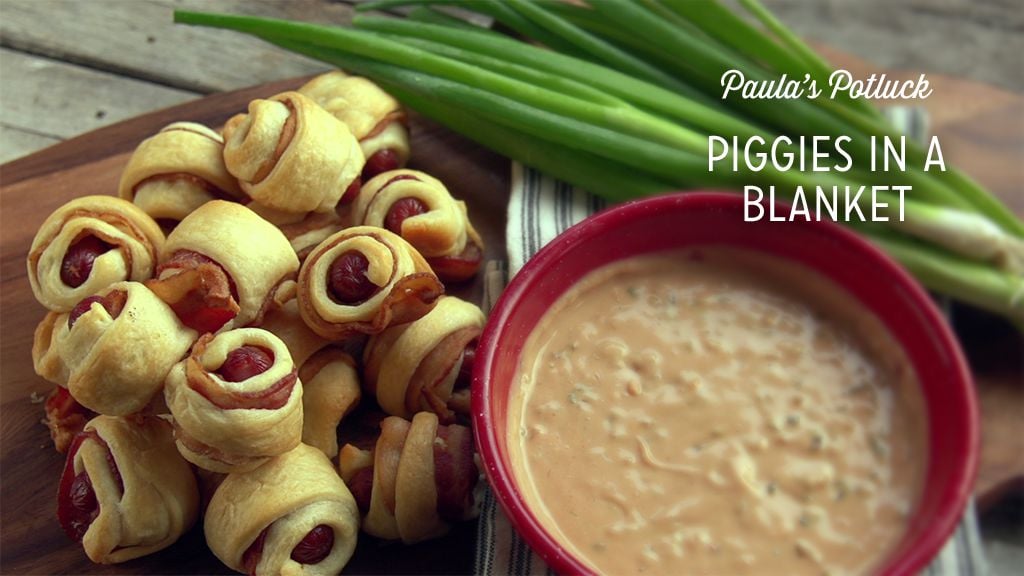This photograph showcases a carefully arranged food display on a wooden table. At the center, we see a cutting board positioned diagonally, adorned with an assortment of dishes. On the left side of the board are "piggies in a blanket," featuring hot dog sausages wrapped in a golden-brown, flaky crust. Adjacent to these, towards the right, is a vibrant red bowl containing a rich, creamy soup, possibly clam or corn chowder, with an orangish-cream hue. Sitting above the bowl, a bunch of fresh green onions with white bulb ends adds a touch of vivid green and white to the composition. Draped across the cutting board on the right, a neatly folded blue and white striped dish towel complements the rustic yet cozy setting. The entire scene is set against a wooden table, creating a warm, inviting atmosphere. The caption "Paula's Potluck: Piggies in a Blanket" clearly indicates the theme of this delectable spread.